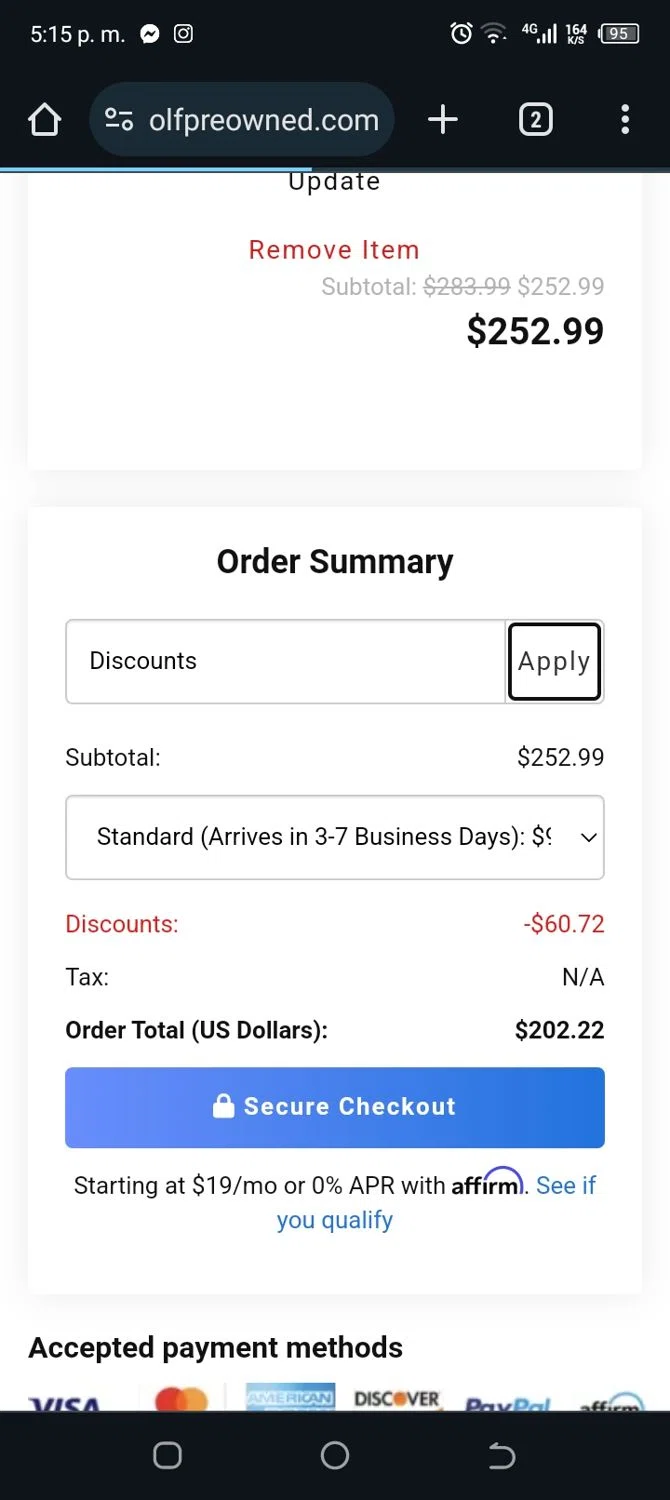This image is a screenshot from the mobile app of olfpreowned.com, displaying an order summary. 

At the very top, there's an "Update" option highlighted in red text, followed by a "Remove Item" link. The subtotal, originally priced at $283.99 (which is crossed out in grey), is now reduced to $252.99, prominently displayed in bold. 

Beneath this, a white box titled "Order Summary" in bold black letters encloses further details. Inside this box are two rectangular sections. The first section mentions "Discounts" with an "Apply" button to the right. Below this, the subtotal is reaffirmed as $252.99 before a dropdown menu indicates "Standard Shipping (3-7 business days)." 

The discount is presented in red, showing a deduction of $60.72. Tax information is marked as "N/A," and the final order total is stated as $202.22 in US dollars. 

At the bottom, there is a blue "Secure Checkout" button alongside an Affirm financing option, which starts at $19 per month with 0% APR. The accepted payment methods listed include Visa, MasterCard, American Express, Discover, PayPal, and Affirm.